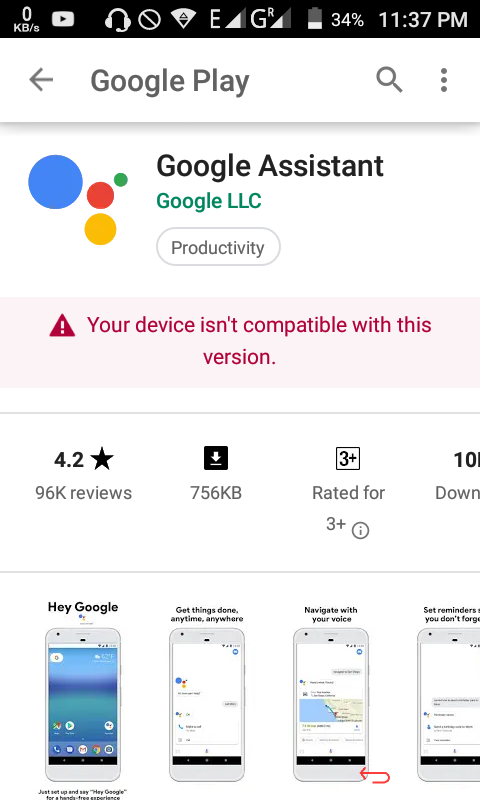The image is a screenshot of someone's Google Play page displayed on a mobile device. At the top, the Google Play icon and text are visible. Below this, the app name "Google Assistant" is prominently featured, with the developer listed as "Google LLC" in green letters. The app is categorized under "Productivity."

To the right, there is a series of four colorful circles arranged vertically: a large blue circle at the top, followed by a slightly smaller yellow circle, a red circle that is smaller still, and a tiny green circle at the bottom. Beneath these circles, a pink box with red text indicates that "Your device isn't compatible with this version," accompanied by a red triangle with an exclamation point.

Further down the page, there are images of four smartphones, each displaying the text "Just set up and say 'Hey Google' for a hands-free experience." Additional promotional text states: "Get things done anytime, anywhere. Navigate with your voice and set reminders so you don't forget."

At the bottom of the screen, the app's rating is shown as 4.2 stars, based on 96,000 reviews. There is also mention of clickable areas for further interactions with the app.

This descriptive and detailed caption comprehensively covers all the visual elements and textual information present in the image.